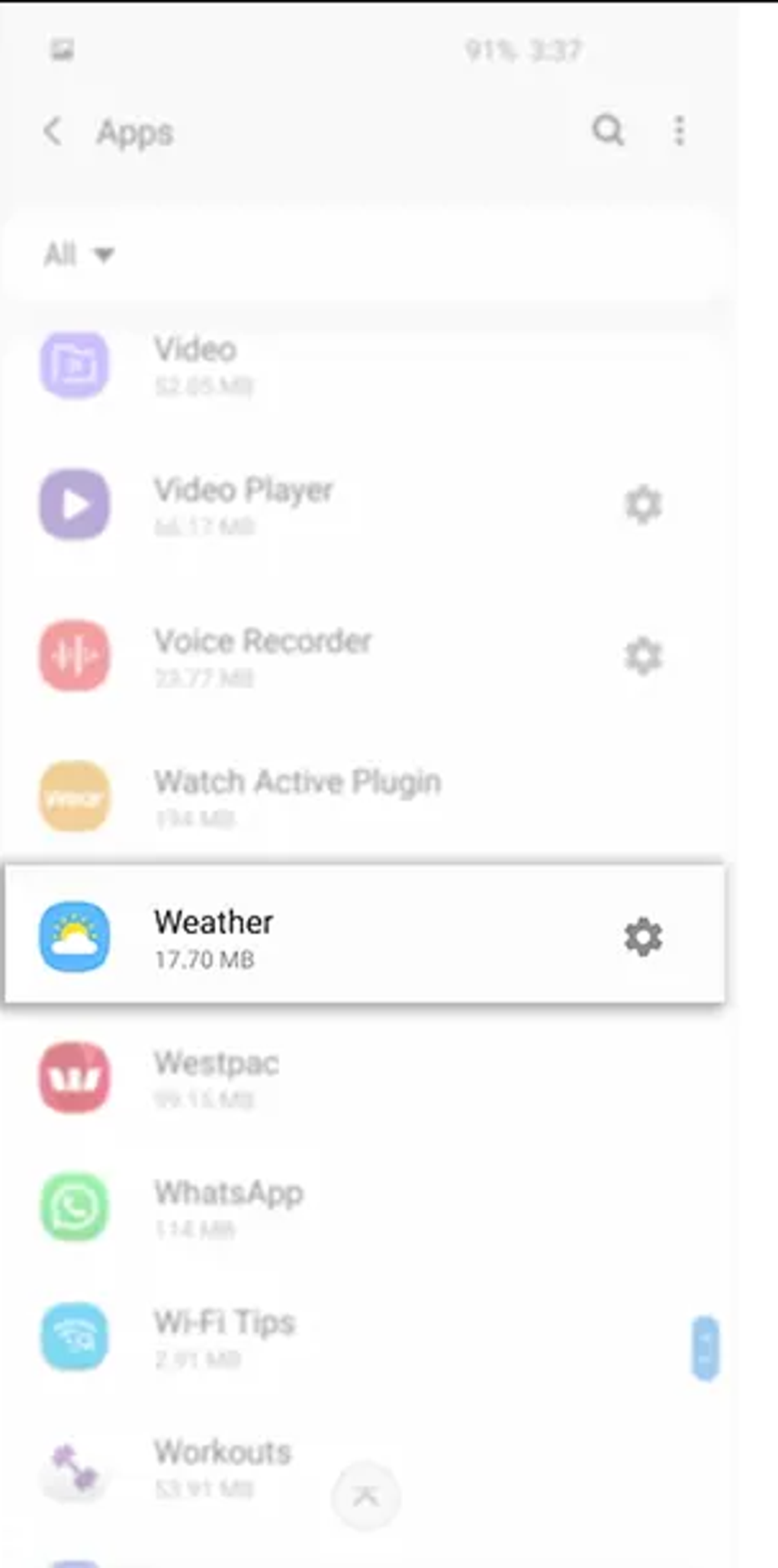The image depicts a section of a smartphone's control panel displaying various apps. The majority of the screen is overlaid with a white filter, rendering the apps nearly invisible, with only faint, blurred outlines and icons of the apps recognizable against a variety of colored backgrounds.

At the top of the screen, there's a narrow, approximately two-pixel black bar that houses several elements: a photo icon, a battery meter indicating 91% charge, the current time displayed as 3:37, a back button, a magnifying glass for search, and a vertical three-dot menu for additional options.

Among the obscured apps, a few are somewhat identifiable despite the white overlay, including app icons and names such as Video, Video Player, Voice Recorder, Watch Again Plugin, Westpac, WhatsApp, Wi-Fi Tips, and Workouts. A scroll button is visible on the right, suggesting that more apps are accessible by scrolling down.

The only app that stands out and is clearly visible is the Weather app. It is housed in a white rectangular frame with a heavy drop shadow making it prominent among the other grayed-out icons. On the left side of this app's icon, there is a graphic— a blue background featuring a sun partially obscured by a cloud with rays of light radiating from it. To the right of this graphic, in black text, the word "Weather" is displayed, with "17.70 MB" written beneath it in gray text. At the far right of the Weather app's tab, there is a gear icon, indicating additional settings or information is available.